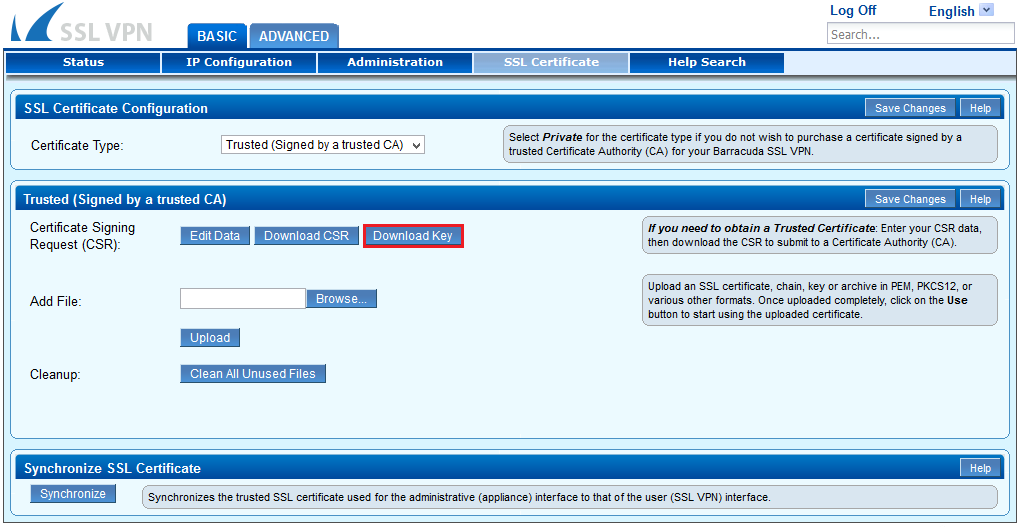Detailed Caption: 

The image displays a desktop application interface for SSL VPN configuration. In the top left corner, "SSL VPN" is labeled in gray. The interface features two tabs, "Basic" and "Advanced," allowing users to switch between different configuration modes. The predominant color scheme consists of shades of blue, with headers such as "Status," "IP Configuration," and "Administration" organizing the various subsections.

Currently, the "SSL Certificate" tab is selected, distinguished by a lighter blue highlight. The main section of the interface is dedicated to "SSL Certificate Configuration," where users can manage certificate types. The selected certificate type is "Trusted," indicating it is signed by a trusted Certificate Authority (CA). There's a note explaining that if users choose "Private" as the certificate type, it implies they do not intend to purchase a certificate signed by a trusted CA for their Barracuda SSL VPN.

Central to the section, the interface highlights options related to the certificate signed by a trusted CA, including "Download Key," "Certificate Signing Request," "Edit Data," and "Download CSR." Users can also browse and upload a file and utilize a "Cleanup" button to remove all unused files.

At the bottom of the interface, a blue "Synchronize SSL Certificate" section includes a "Synchronize" button, which is set to synchronize the trusted SSL certificate used for the administrative interface of the SSL VPN.

The interface also features options for logging off and changing the language, as indicated by the "Log Off" button and "English" label. The overall visual presentation is a mix of baby blue and darker blue, suggesting a cohesive design for use on Windows or potentially mobile platforms.